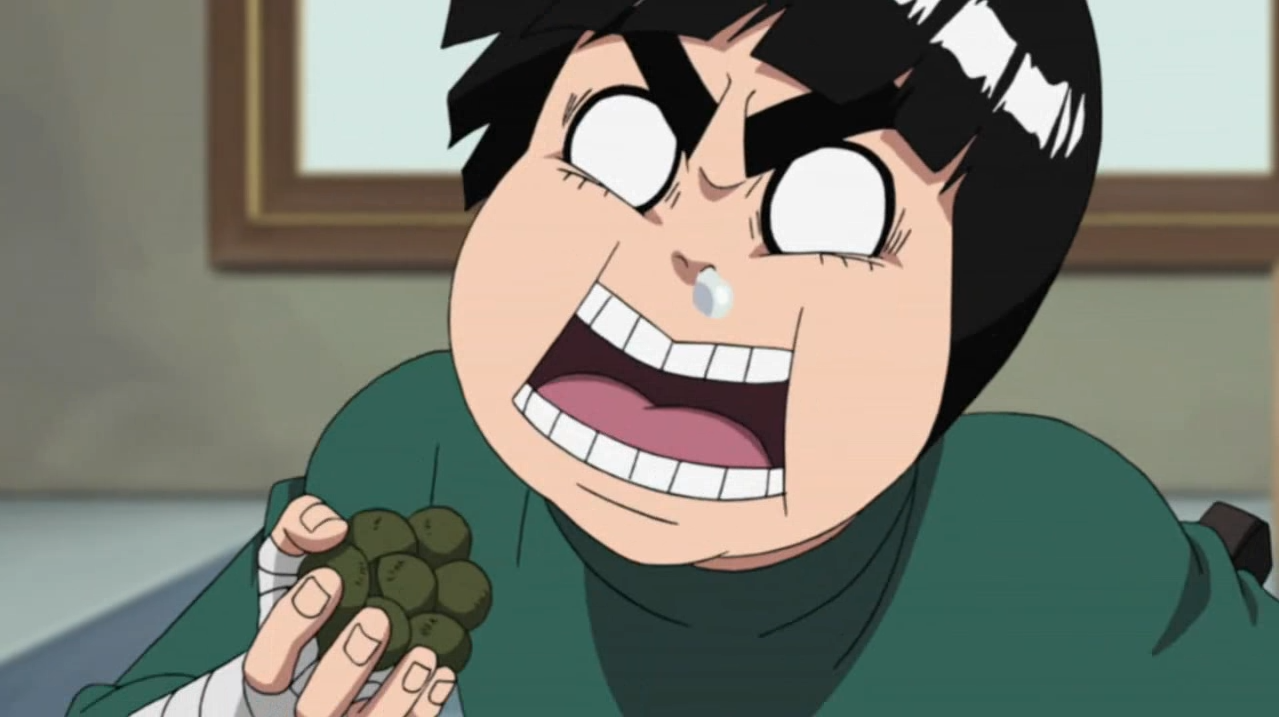This is a close-up anime image depicting a person in a state of intense anguish or anger, characterized by exaggerated facial expressions. The individual has short, shiny black hair, thick eyebrows furrowed in a V shape, and large eyes completely whited out with black liner. They are wearing a green garment visible from the upper chest. A white bandage wraps around their hand, leaving only the tips of their fingers exposed as they clutch a fistful of small, round green objects, possibly berries or olives. The person's mouth is wide open, revealing their teeth and pink tongue, and there is a noticeable droplet, possibly snot, hanging from their nose. The background is simplistic, featuring a wall with a brown wooden frame partially outlining what could be a window or picture.